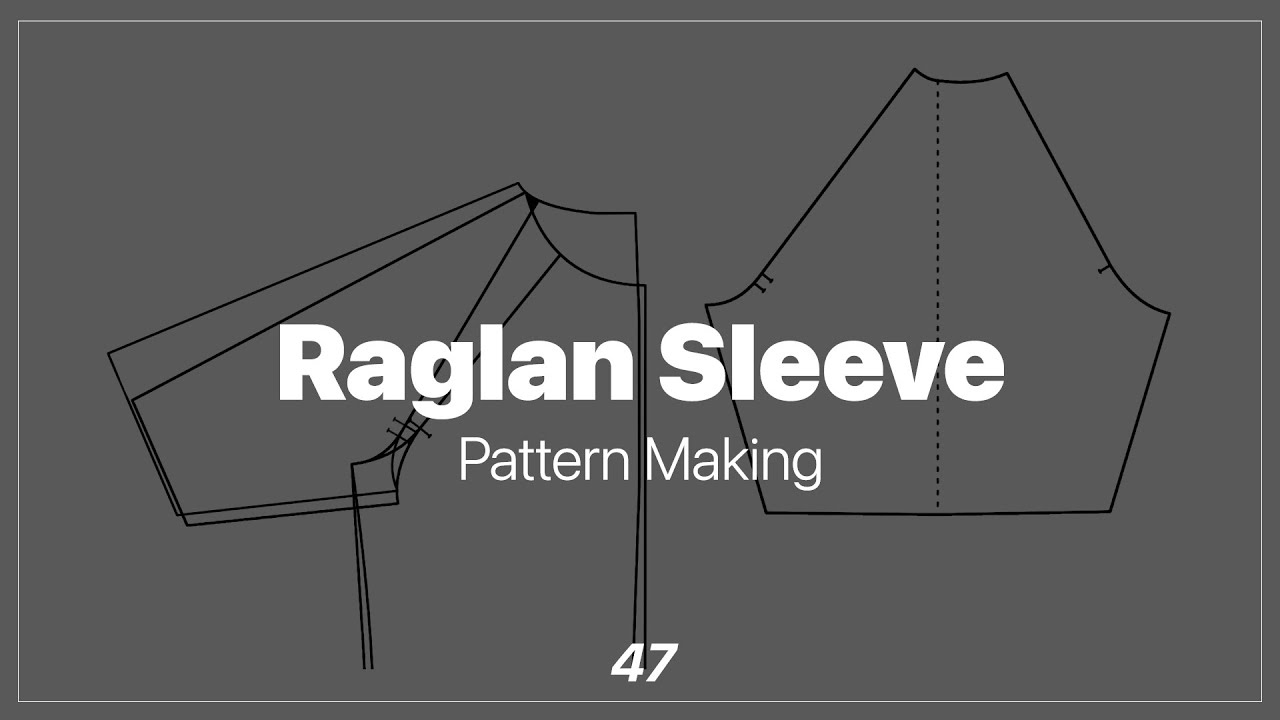The image is a slide title for an "Episode 47 Raglan Sleeve 1 Pattern Making Tutorial." The background features a tan gradient transitioning to white from left to right. The slide has black text with the title prominently displayed in bold letters. Positioned to the right of the text, there is a detailed sleeve template sketch, marked with different colored lines (dark blue, lighter purple, and green) to indicate various cut-out points and pivot lines. The diagram appears to be instructional, aimed at illustrating the initial steps of creating a Raglan sleeve pattern.